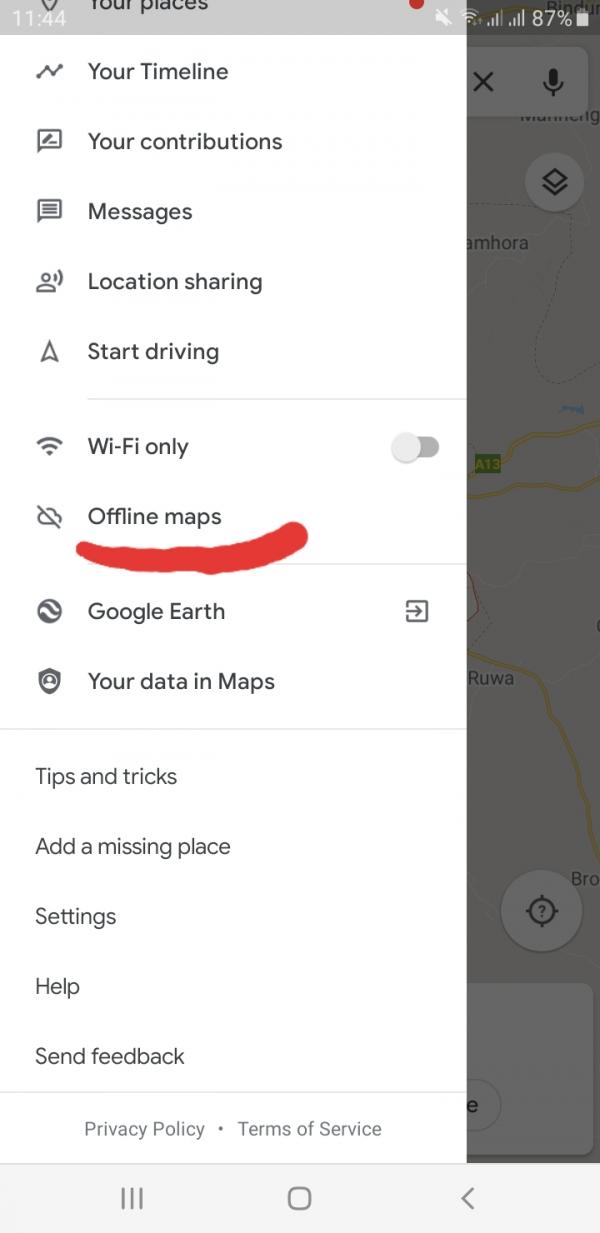The image depicts an options menu from a Google application, likely Google Maps. The interface shows a semi-transparent map displayed as the background, with a standard taskbar at the top displaying time, battery life, and other system indicators. At the bottom, there is a menu bar featuring a central button that grants access to the main menu.

A prominent white sidebar menu is visible on the left side, containing various settings and options, distinguished by gray lines for separation and accompanied by icons next to each text line. At the top, the menu includes items such as "Your places," "Your timeline," "Your contributions," "Messages," "Location sharing," and "Start driving."

The menu continues with a section featuring a switch for "Wi-Fi only" mode and an option for "Offline maps," which has been underlined in red, indicating an edit to this screenshot and not part of the original interface. Below this are more sections demarcated by additional lines, containing items like "Google Earth" and "Your data in Maps," followed by "Tips and tricks," "Add a missing place," "Settings," "Help," and "Send feedback."

At the very bottom of the menu, there are links to the "Privacy policy" and "Terms of service."